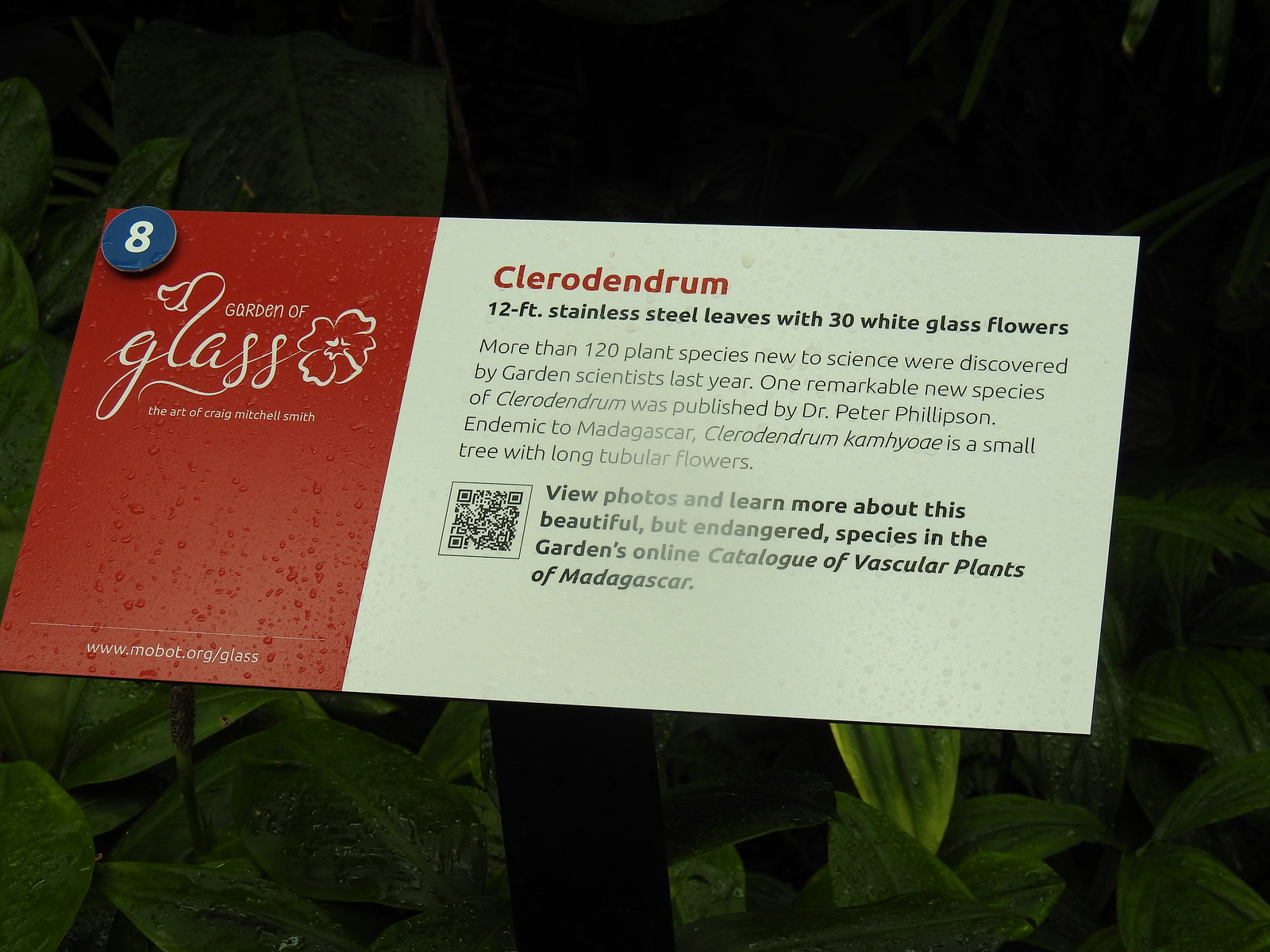The image captures a detailed outdoor scene featuring a vibrant nature setting with abundant green leaves and various plants in the background. Prominently displayed in the foreground is a nature sign mounted on a black stand, which could be either wooden or metal. The sign itself has a distinct design: the left third is red with white text, reading "Garden of Glass" with the words "The Art of Craig Mitchell Smith" and a website at the bottom. Adorning the top-left corner of the sign is a circular blue emblem with a white number 8 in its center.

The right side of the sign features a white background with a detailed description of a piece titled "Cleodendron." Emphasized in red text is the title, followed by black text that describes "12-foot stainless steel leaves with 30 white glass flowers." The accompanying paragraph provides additional information about the plant species and their discovery, mentioning that over 120 new species were identified by garden scientists last year. Among these was a remarkable new species of Cleodendron, documented by Dr. Peter Philipson and endemic to Madagascar, known as Cleodendron cameoae, a small tree with long tubular flowers. The sign encourages viewers to learn more about this endangered species through the garden's online catalog. At the bottom of the sign, a QR code is provided for accessing photos and further details.